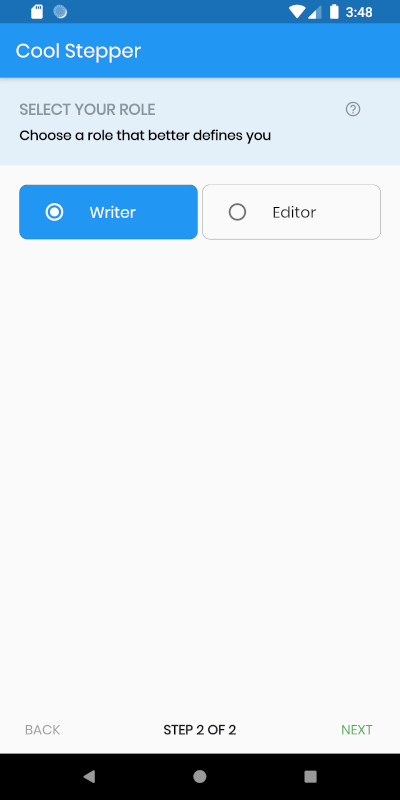The image displays a webpage on a mobile phone. The screen shows a time of 3:48, a fully charged battery, and a Wi-Fi connection. At the top of the webpage, there is a blue header and background with the text "Cool Stepper" written in white letters. Below this, a gray box with bold black text reads, "Select Your Role. Choose a role that better defines you." A question mark inside a circle is also present, possibly indicating help or additional information.

Immediately beneath the instruction, there are two role options: "Writer" and "Editor." The "Writer" option is highlighted with a blue background and white text, indicating it is selected, while the "Editor" option is displayed with black text on a white background inside a black-bordered box. 

Further down, at the very bottom of the page, "Back" is written in small letters. Above this, it states "Step 2 of 2" in bold black letters, indicating the current step in the process. Next to this, there is a "Next" button in small green capital letters.

At the very bottom of the mobile screen, there are three icons in gray: a triangle, a circle, and a square. The footer of the phone is entirely black. Additionally, at the top of the webpage, there are two small icons, a circle, and a square, whose purposes are unclear.